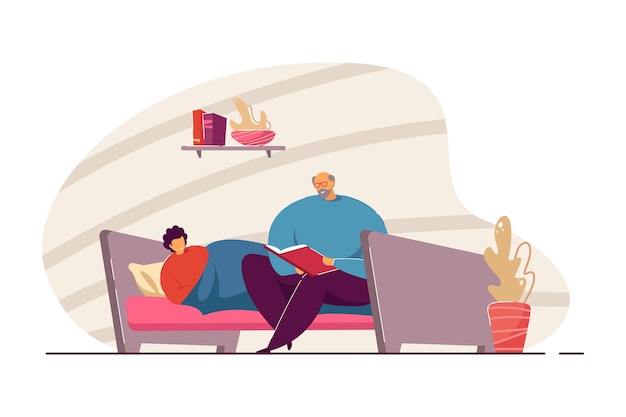The stylized illustration depicts a bedroom scene with a man reading a book to a person lying in bed. The background features a beige and off-white striped pattern. On the wall above the bed, there is a shelf holding two books, one orange-red and the other purple, alongside a red vase with beige and yellowish-gold plants. The bed itself is a purplish-gray color, dressed in a pink mattress and a medium blue blanket. The person in bed, who appears to be male, has black curly hair and wears a red sweater. He rests against a beige pillow. Sitting on the bed beside him is an older man with a bald head, gray side hair, and a gray beard, adorned with red glasses. This man wears a turquoise sweatshirt and dark purple pants, and he's holding an open, reddish-purplish book. To the right of the bed, there's another potted plant in a red pot with yellowish-gold foliage.